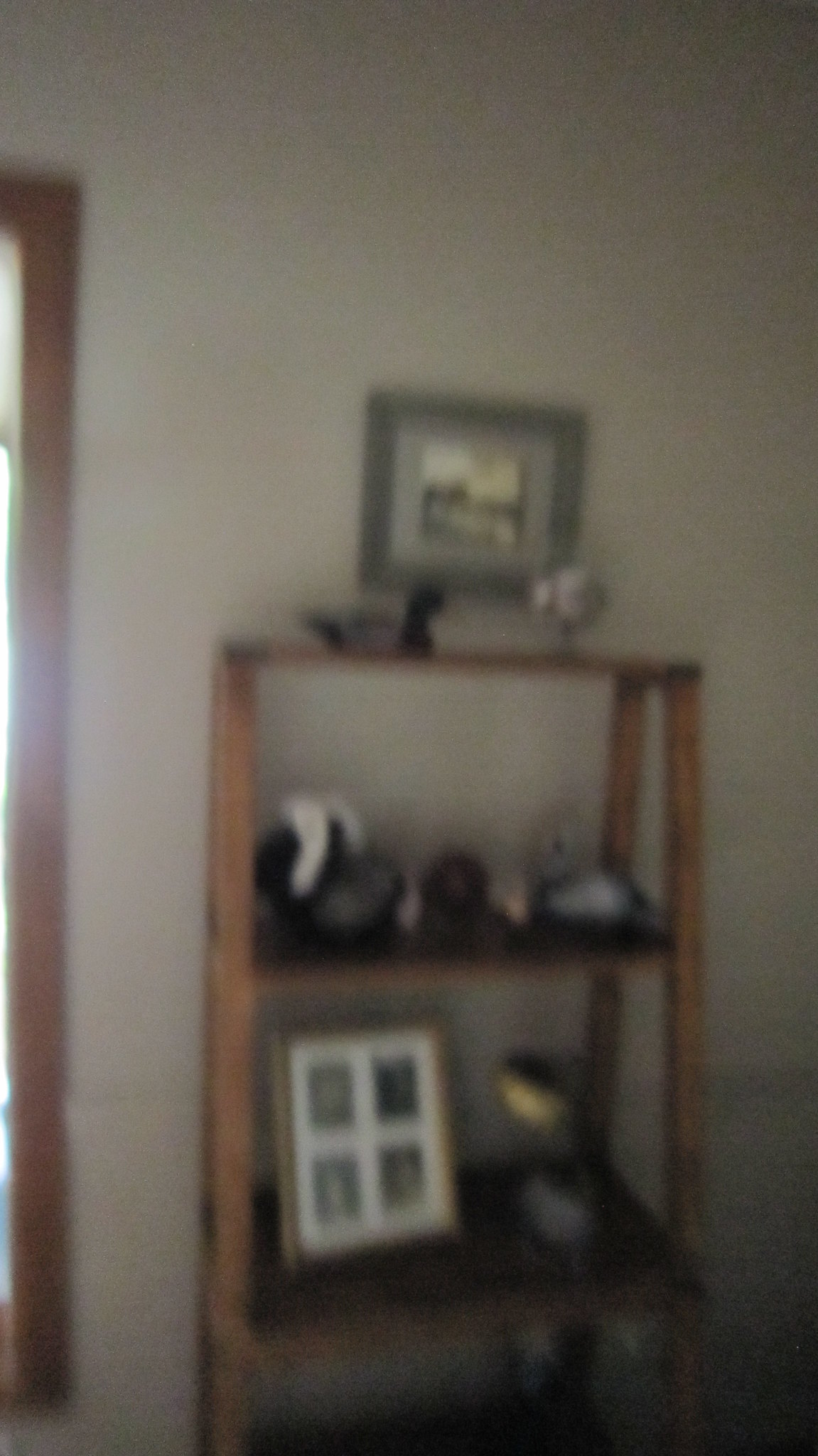This photograph, slightly blurred, captures a simple yet detailed interior scene. A gray wall serves as the backdrop, against which a dark brown wooden door frame is positioned. An open wooden shelving unit, standing prominently to the right of the door frame, features three shelves. Above the shelves, a framed picture with a dark gray border and a light gray matting hangs on the wall, depicting a serene landscape of sky and trees. The top shelf holds a ceramic duck figurine and an empty glass, adding a touch of whimsy. On the bottom shelf, a multi-picture frame displays four distinct images, adding a personal touch to the setting.